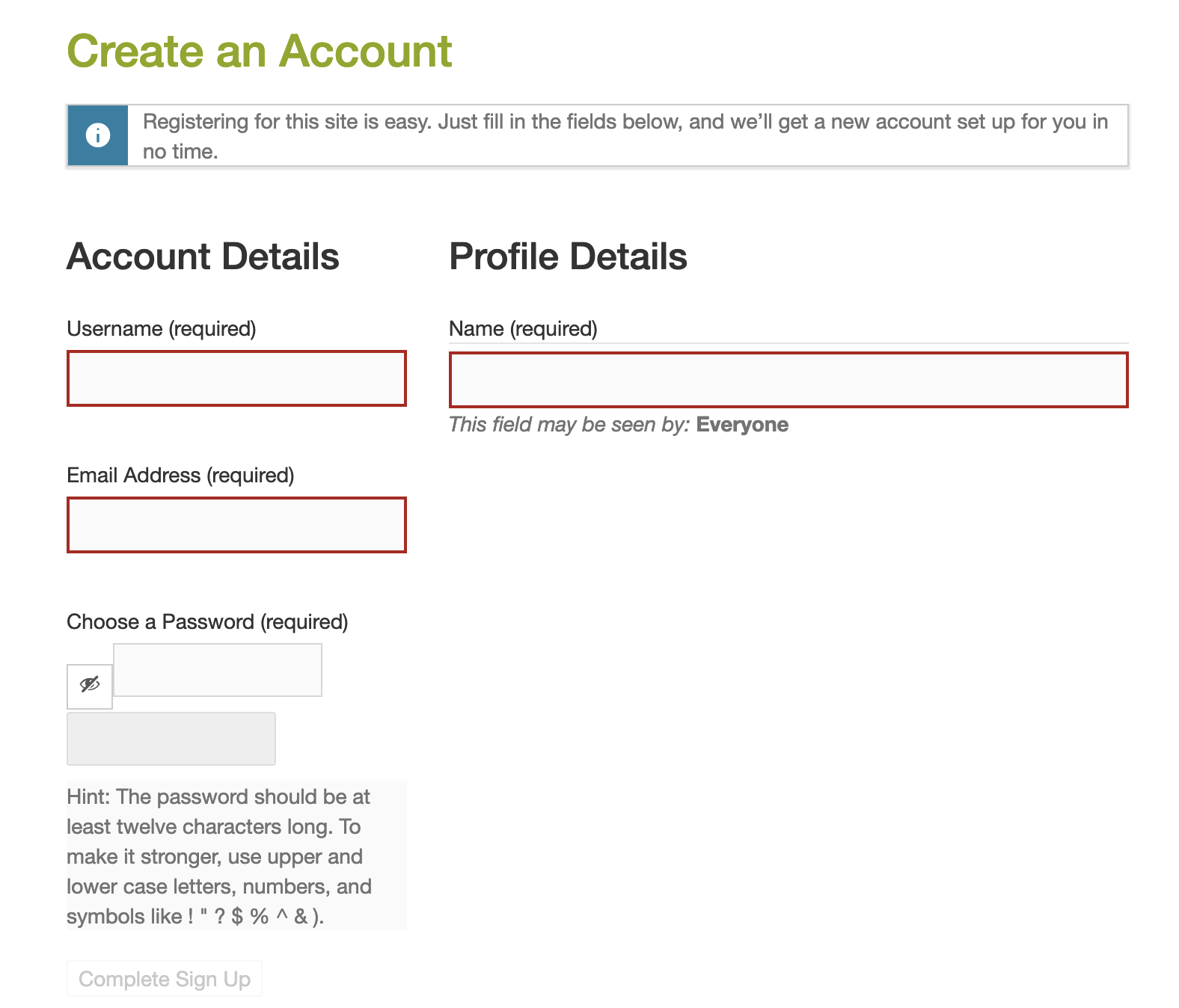The image is a screenshot of a website's sign-up page. At the very top, in green text, it prominently displays the phrase "Create an Account." Directly beneath this, an information bar with a cyan-colored information icon (a lowercase "i" within a circle) informs users: "Registering for the site is easy. Just fill in the fields below and we'll get a new account set up for you in no time."

The sign-up form is divided into two columns. The left column, labeled "Account Details," includes the following required fields: 
1. Username
2. Email Address
3. Choose a Password
   - Below the password field, a hint advises: "The password should be at least 12 characters long. To make it stronger, use upper and lowercase letters, numbers, and symbols like: ! " ? $ % ^ &."

At the bottom of this column is the "Complete Sign-Up" button, which is currently faded out (indicating it is inactive) due to the unfilled fields, which are highlighted in red to signify they are required.

The right column, labeled "Profile Details," contains a single field for entering a name, also marked as required. Below this field, a note in bold emphasizes: "This field may be seen by everyone."

The overall design is minimalist, with a completely white background and predominantly black text. The green text and cyan icon provide subtle color accents, creating a clean and straightforward user interface.